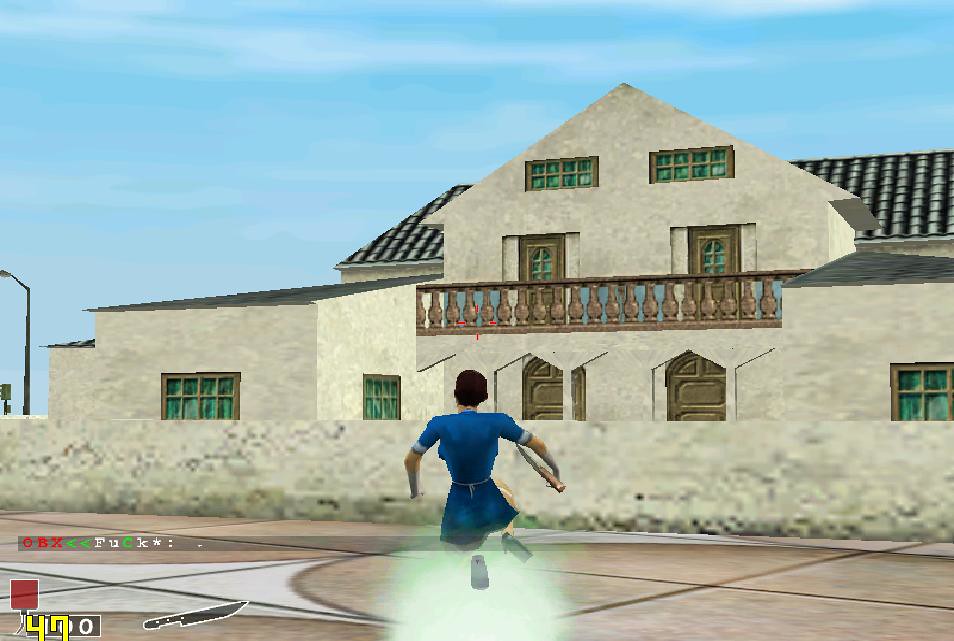In this screen capture from a rare, early 2000s video game, a female character is depicted sprinting towards a two-story building while wielding a knife in her right hand. The character's weapon is also shown as an icon in the bottom left corner of the screen. The two-story building ahead features several architectural elements, including a wall, multiple windows, a roof, a balcony, and four doors. The setting is under a vibrantly blue sky, adding a contrast to the intense action unfolding in the scene.